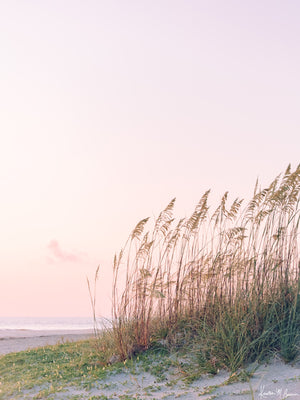In this photograph of a beach scene, we see an expansive view of softly lit sand extending across the foreground, creating a beautiful and serene sandy surface. The lower right corner showcases tall beach grass bending in the wind, its green bases transitioning to brown tips, indicative of the changing season. Taller reeds and various grassy vegetation, including low-cut grass and beech grass, spread out towards the ocean, adding texture and depth to the scene. To the left, the sky appears overcast with a hint of pink from the setting sun, barely allowing the surface of the water to be discernible. A small wave approaches the shore, capped with white foam, further enriching the coastal landscape. The photograph also includes a subtle watermark in the bottom right corner, serving as the photographer’s signature. This meticulously detailed image perfectly captures the tranquil, windswept beauty of a natural beach environment.